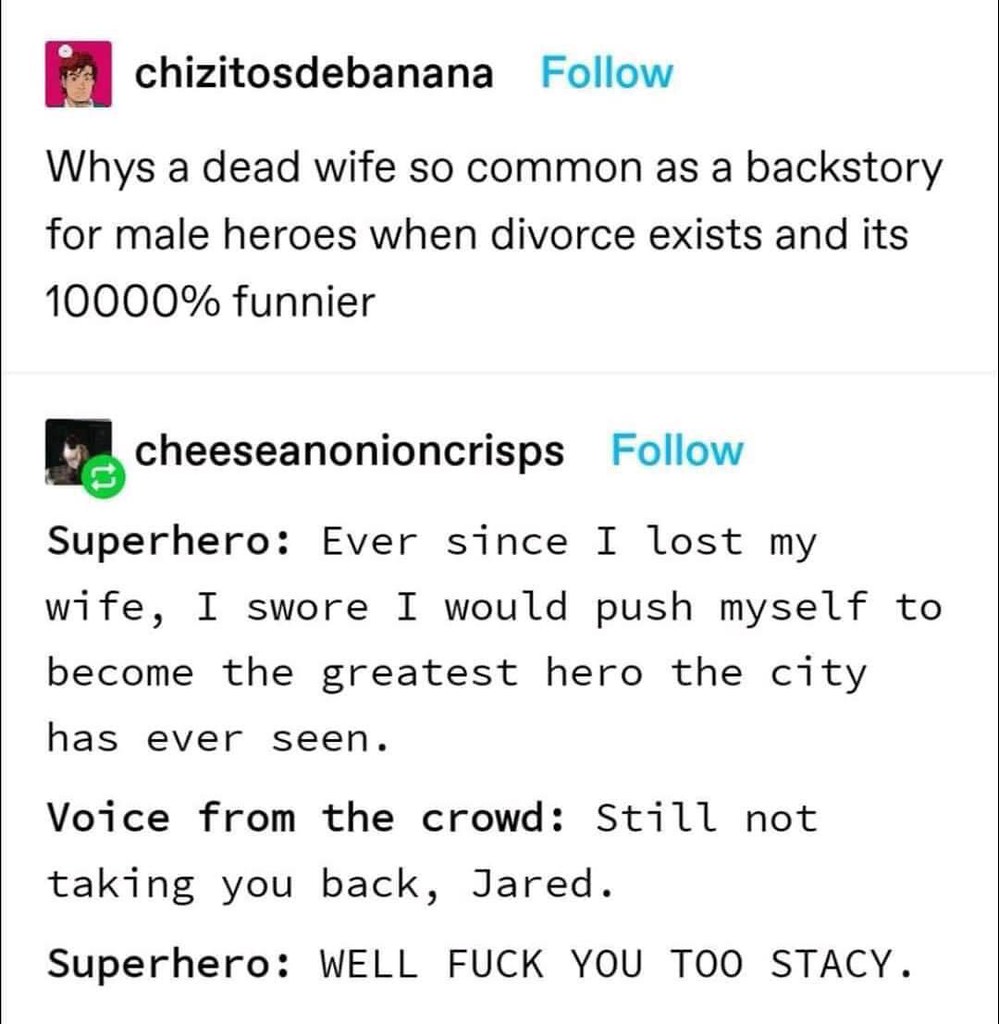This vertical-rectangular image appears to be a screenshot of a social media post with user comments. The top post is by Chizitos de Banana, identified by an avatar showing a pink rounded rectangle with a man with reddish hair. His comment questions, "Why is a dead wife so common as a backstory for male heroes when divorce exists, and it's 10,000% funnier?" Below this, Cheese and Onion Crisps replies, embodying a superhero: "Ever since I lost my wife, I swore I would push myself to become the greatest hero the city has ever seen." A following comment humorously cuts in with, "Voice from the crowd: still not taking you back, Jared," to which the superhero character responds, "Well, fuck you too, Stacy."